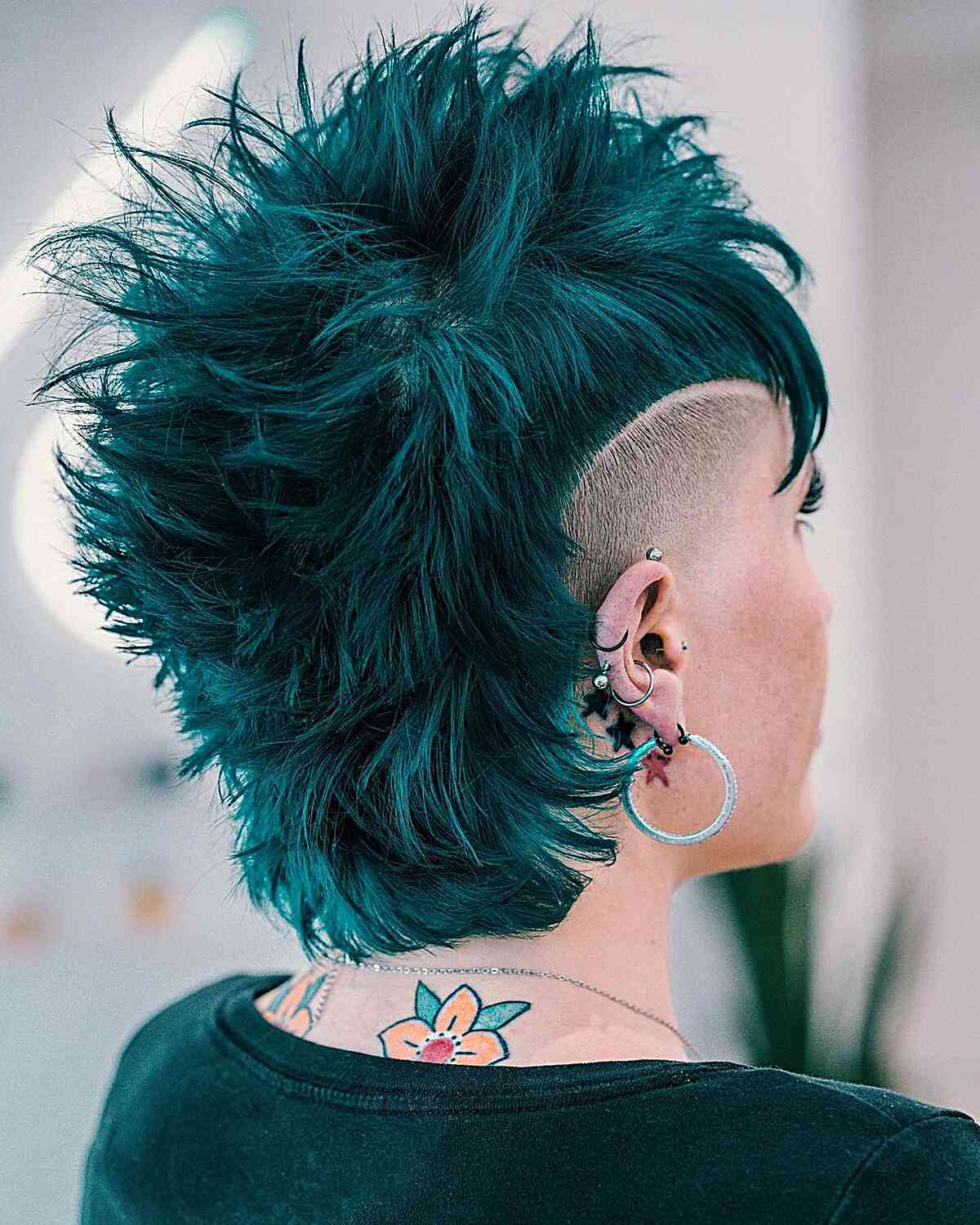The full-color photograph, taken indoors during the day possibly using natural light, features a young Caucasian woman with a striking punk hairstyle, viewed from behind. Her hair, dyed an intricate blend of gray, bluish-gray, and aqua blue with a greenish tint, flows messily in a thick, vibrant mohawk, while the sides of her head are shaved in a curved arch and feature thin black hair. She is adorned with multiple piercings: a large silver hoop earring, several smaller steel studs, three clamped earrings, and a ball earring at the top of her ear. Behind her ear, there are three star tattoos—two black and one red. The back of her neck displays two tattoos of yellow flowers with red centers and green leaves. She is dressed in a simple black crew neck t-shirt. The background of the image is a blurred wall, highlighted by spots of sunlight in the upper left corner and a few patches of blue, red, and gold in the lower left.